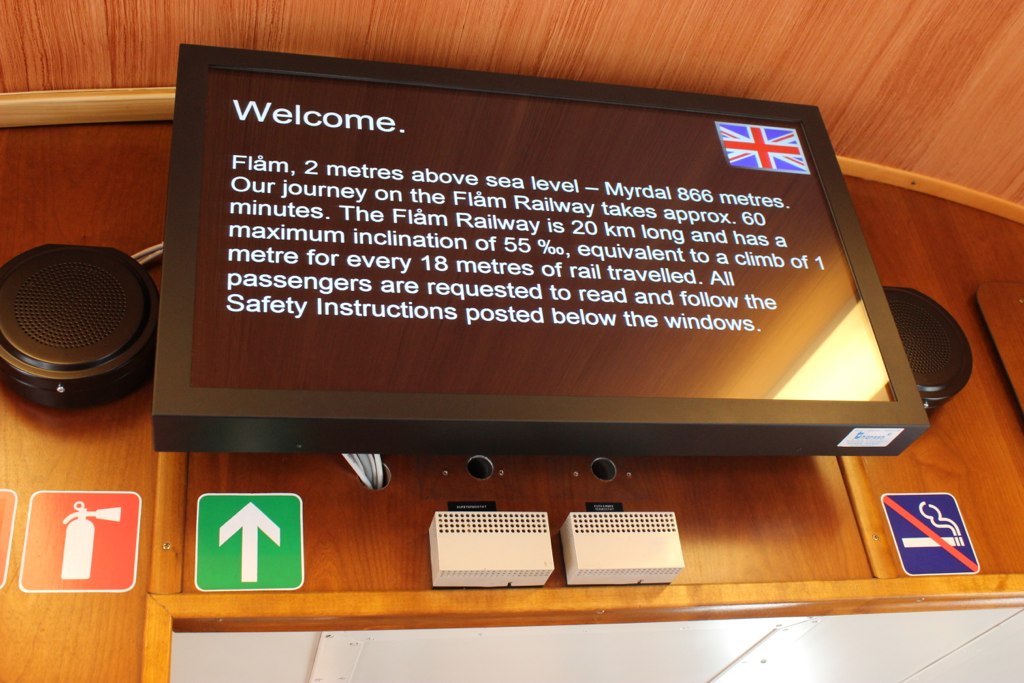This image captures an elegant wood-paneled interior of a Flom Railway train, highlighting a centrally-mounted black flat screen television against a darker wood wall. Flanking the TV on either side are round, black speakers. The welcoming message on the screen reads: "Welcome, Flom, 2 meters above sea level, Myrtle, 866 meters. Our journey on the Flom Railway takes approximately 60 minutes. The Flom Railway is 20 kilometers long and has a maximum inclination of 55%, equivalent to a climb of 1 meter for every 18 meters of rail traveled. All passengers are requested to read and follow the safety instructions posted below the windows." Additionally, a British flag icon is visible at the top right corner of the screen. Below the TV, various safety signs are displayed, including a red fire extinguisher symbol, a green upward-pointing arrow, and a blue no-smoking sign. The ceiling above is adorned with light brown wood panels, with visible wood grain enhancing the cozy ambiance. Overall, the color scheme within the image encompasses shades of brown, black, red, green, and blue, collectively contributing to a warm, inviting atmosphere inside the train.